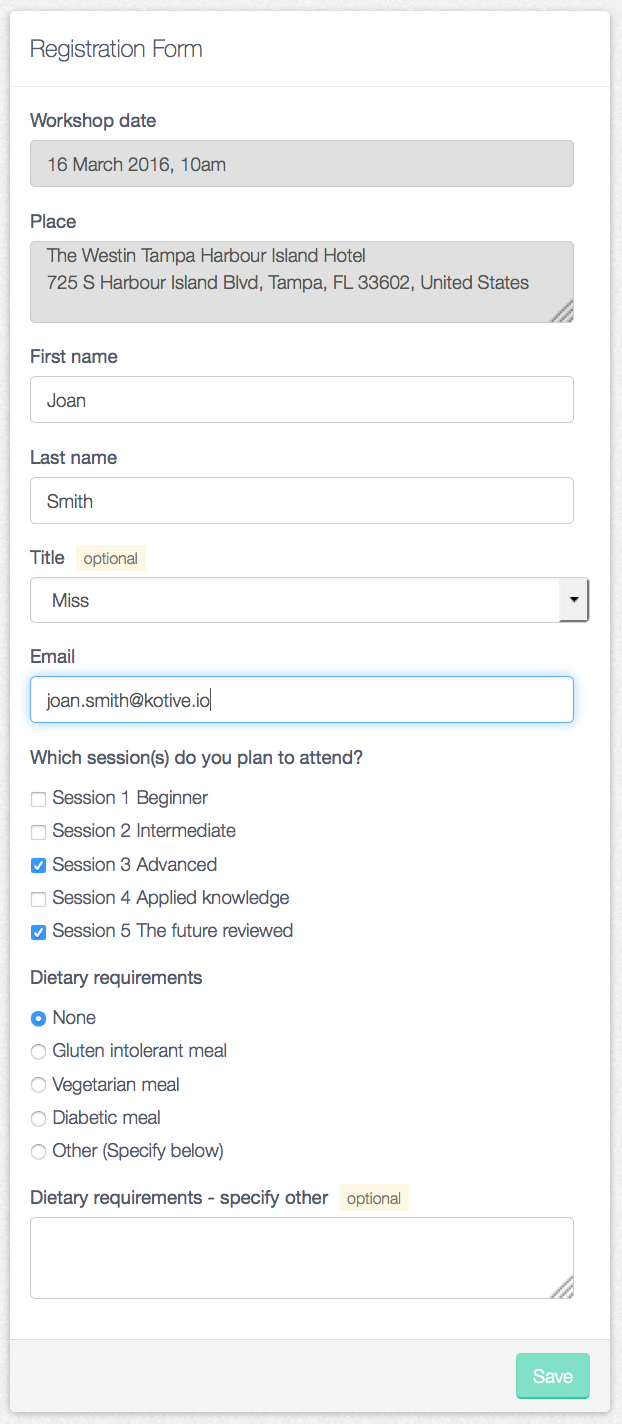The image depicts a detailed registration form with a white background and a gray outline, appearing quite tall and longer than a typical portrait mode image. 

At the very top, the form is titled "Registration Form," followed by a thin gray line. Below this, the following information and sections are presented sequentially:

- **Workshop Date**: Displayed in a gray rectangular box.
- **Place**: The address is also shown in a gray rectangular box.
- **First Name**: The name "Joan" is filled in a white box.
- **Last Name**: The surname "Smith" appears in another white box.
- **Title**: Marked as optional with a yellow highlight, featuring a dropdown menu that currently shows "Miss."
- **Email**: The email address field is filled in a white box, which is distinctly highlighted with a blue glow.

Below the personal information section, the form includes a session selection area titled "Which sessions do you plan to attend?" Here, five checkbox options are listed:

1. Session One: Beginner
2. Session Two: Intermediate
3. Session Three: Advanced (checked)
4. Session Four: Applied Knowledge
5. Session Five: Future Review (checked)

Following the session choices, there's a section for dietary requirements with checkboxes. The options provided include none, gluten intolerant meal, vegetarian meal, diabetic meal, and other specified below. The "None" option is the only one checked. Additionally, there's a prompt to specify other dietary requirements, marked as optional and highlighted in yellow, with a white text box provided for entering details.

Finally, at the bottom right corner of the form, there is a green "Save" button with the text written in white.

Overall, the image is comprehensive and visually organized, allowing for clear input of registration information and preferences.